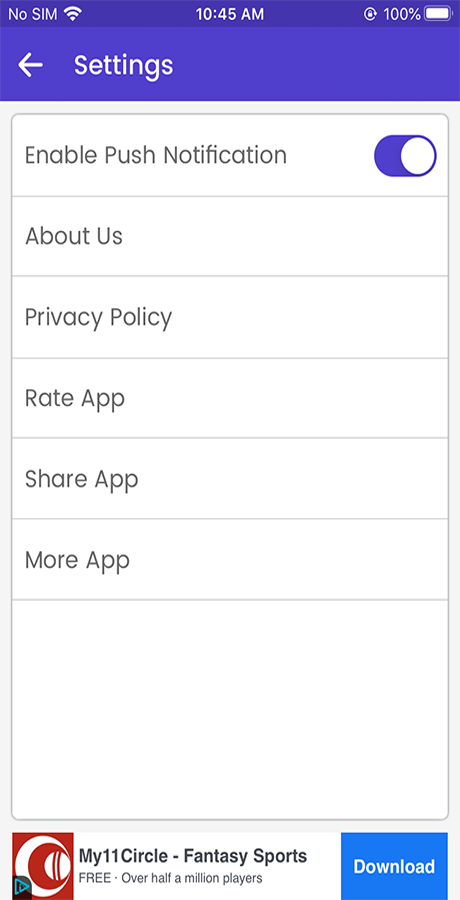This is a screenshot of the settings page from a mobile application. At the top left corner, there is a white back button accompanied by the word "Settings" in white text, all set against a purple background which occupies about one-tenth of the entire screen. Below this header, the settings options are presented on a white background with each option separated by grey lines.

1. The first option reads "Enable Push Notification," featuring a toggle switch on the right side that is currently slid to the right, indicating that push notifications are enabled.
2. The second section is labeled "About Us."
3. The third option displays "Privacy Policy."
4. The fourth option is "Rate App."
5. The fifth says "Share App."
6. The final option at the bottom of this list reads "More App."

At the very bottom of the page, there's an advertisement section showing an ad with a red logo on the left. The ad text includes "My 11 is so cool" in bold black font, followed by "Fantasy Sports." Beneath this, a line of grey text states "Free, over half a million players." In the bottom right corner of the ad, there is a blue button with white text that says "Download."